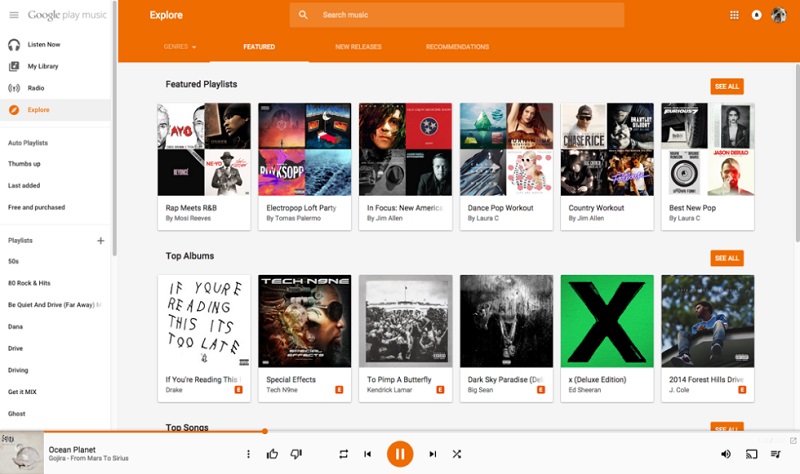The image showcases a detailed view of a web interface, specifically for Google Play Music. 

At the very top left corner, there is a vertical stack of three horizontal lines, commonly known as a hamburger menu. Adjacent to this menu icon, the Google Play Music logo is prominently displayed. Beneath the logo, there are three small black icons representing different user options.

To the right of these icons, a series of navigation tabs are listed: "Listen Now," "My Library," and "Radio." Following these, an orange-highlighted tab reads "Explore," signaling its active selection. Subsequent to the "Explore" tab, four additional navigable tabs are available.

In the center, a large search bar is positioned prominently. To its right, a user profile picture featuring a bulldog is visible, next to a white circle containing a black triangle, possibly indicating a play button, and a grid icon made up of white dots.

Below the "Explore" section, there are subcategories such as "Genres," "Featured," "New Releases," and "Recommendations," all displayed in white text against the interface's general layout.

Toward the bottom, on the left side, "Featured Playlists" is highlighted within a white-bordered section. Here, six playlists are arranged horizontally, each displaying a collage of four album covers. The first playlist is titled "Rap Meets R&B," featuring well-known artists like Neo, Ayo, and Usher. Although the name of the creator is too blurry to discern, this format repeats for six different playlists.

Further down is a section titled "Top Albums," which also displays six album covers arranged horizontally across the interface.